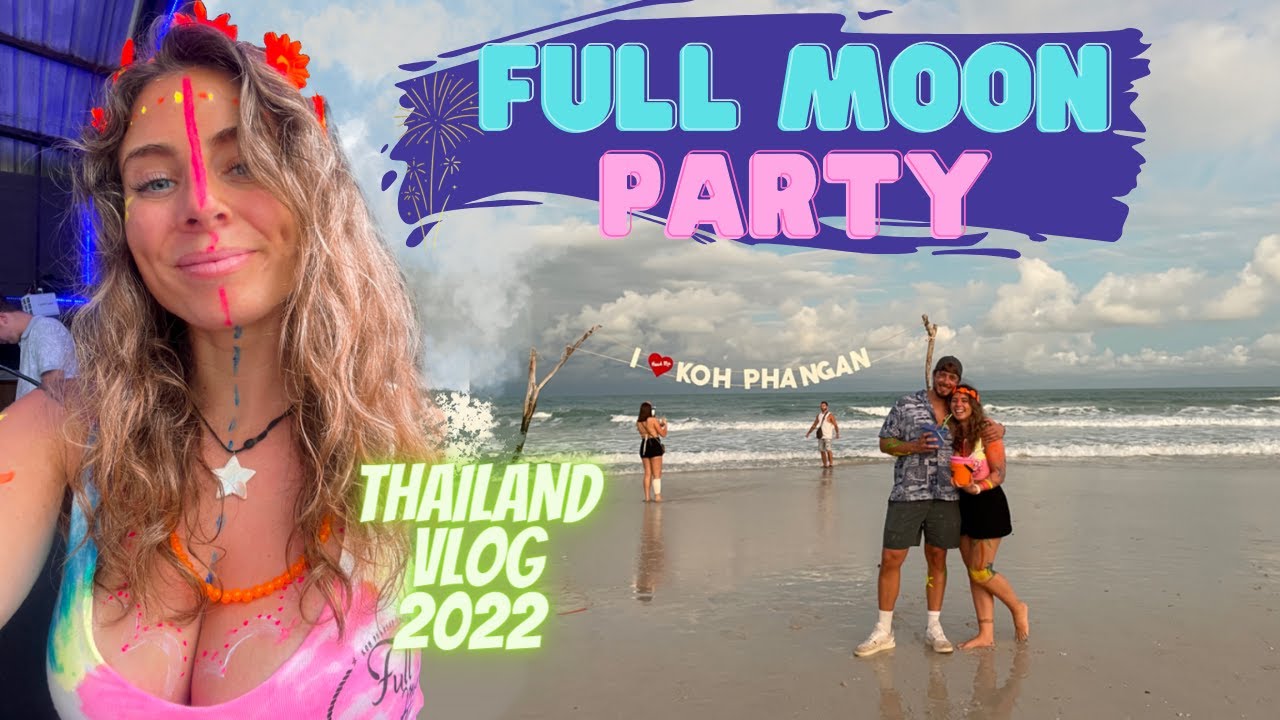The image is a vibrant promotional shot, possibly for a party advertisement or a travel vlog. On the left-hand side, a Caucasian woman with long, flowing dirty blonde hair is featured in a selfie. She wears an orange headband adorned with flowers and an orange beaded necklace, complemented by a black rope with a white star pendant. Her face is elaborately painted with pink lines, yellow dots, and a green stripe running down the center to her chest, highlighting her cleavage. On the right-hand side, there is a lively beach scene under a large blue sky with clouds. Here, the same woman stands with a man who has his arm around her; they are smiling with the ocean waves splashing behind them. In the background, two other people are partially visible behind a blue banner featuring colorful fireworks. The text on the banner reads "Full Moon Party," and underneath it, "Thailand Vlog 2022."